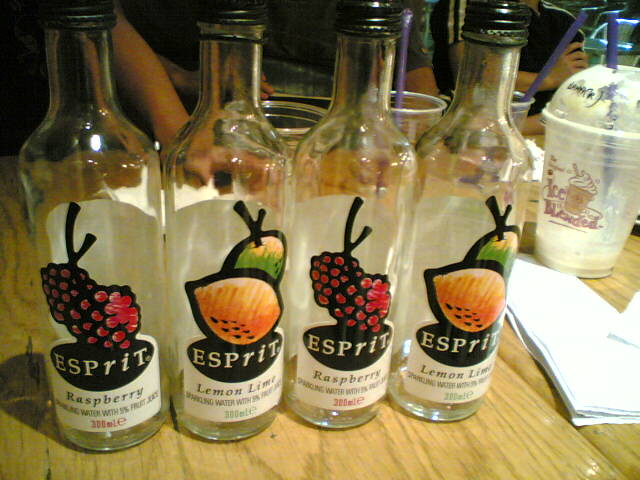In the image, there are four empty glass bottles of ESPRIT sparkling water lined up on a light laminate wood table. From left to right, the flavors are raspberry, lemon-lime, raspberry, and lemon-lime. Each bottle features a vibrant illustration of the respective fruit: the raspberry bottles display two raspberries, and the lemon-lime bottles show a lemon and a lime. The ESPRIT logo is written in white letters with the 'R' and 'I' in lowercase and italicized, placed above the flavor name and milliliter content. Behind the bottles, there are three clear plastic cups; two have purple straws, and the one on the far right has a blue straw and features the text "ICE BLENDED," suggesting it held a frozen drink. To the right of the bottles, there is a stack of white napkins. In the background, the partial image of a white person's hand is visible, and there are multiple blurry figures suggesting a busy environment, possibly a drink shop.